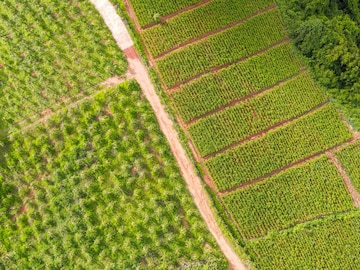This aerial photograph showcases a divided agricultural landscape bisected by a prominent white dirt road running vertically from the top to the bottom of the image. On the left side of the road, several vertical rows of light green treetops are visible, suggesting deliberate cultivation. These rows extend from the top left corner down to the bottom of the image. On the right side of the road, the terrain is divided into multiple horizontal rows likely used for planting crops, interspliced with dirt paths arranged at a slight diagonal towards the upper right corner. The top right corner of the image is filled with dense greenery, probably trees, contrasting with the orderly rows of crops below. The photograph is small and rectangular, presenting this structured patchwork of varying greens and pathways, indicative of a well-planned agricultural area.